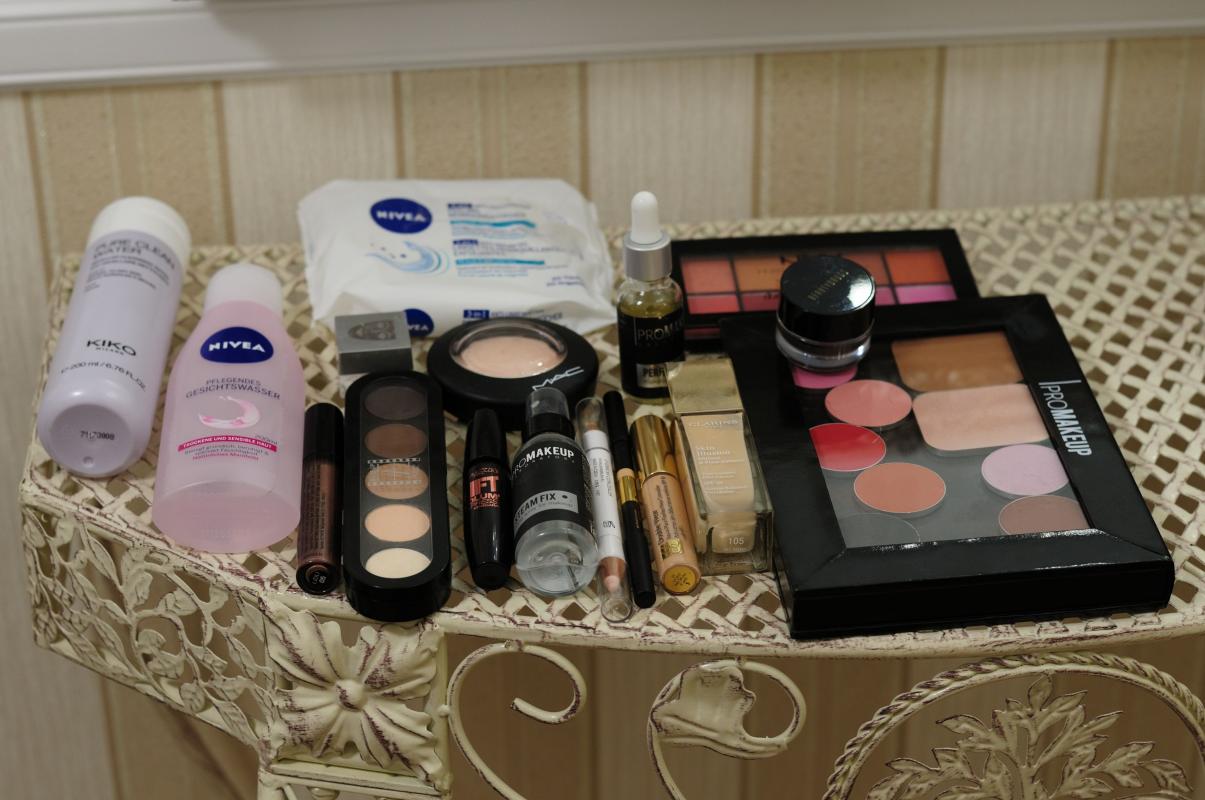This photograph features an assortment of makeup products arranged on a decorative metal lattice table. The table's intricate floral designs frame the collection, adding an elegant touch to the scene. The assorted items include numerous eyeshadow palettes in a variety of colors, a selection of lipsticks, bottles of foundation, sprays, eyeliners, and mascaras. Also present are skin concealer palettes, a compact with powder, alongside practical items such as wet wipes and makeup removing solution. The setup suggests a comprehensive and well-organized makeup kit, ideal for creating various looks.